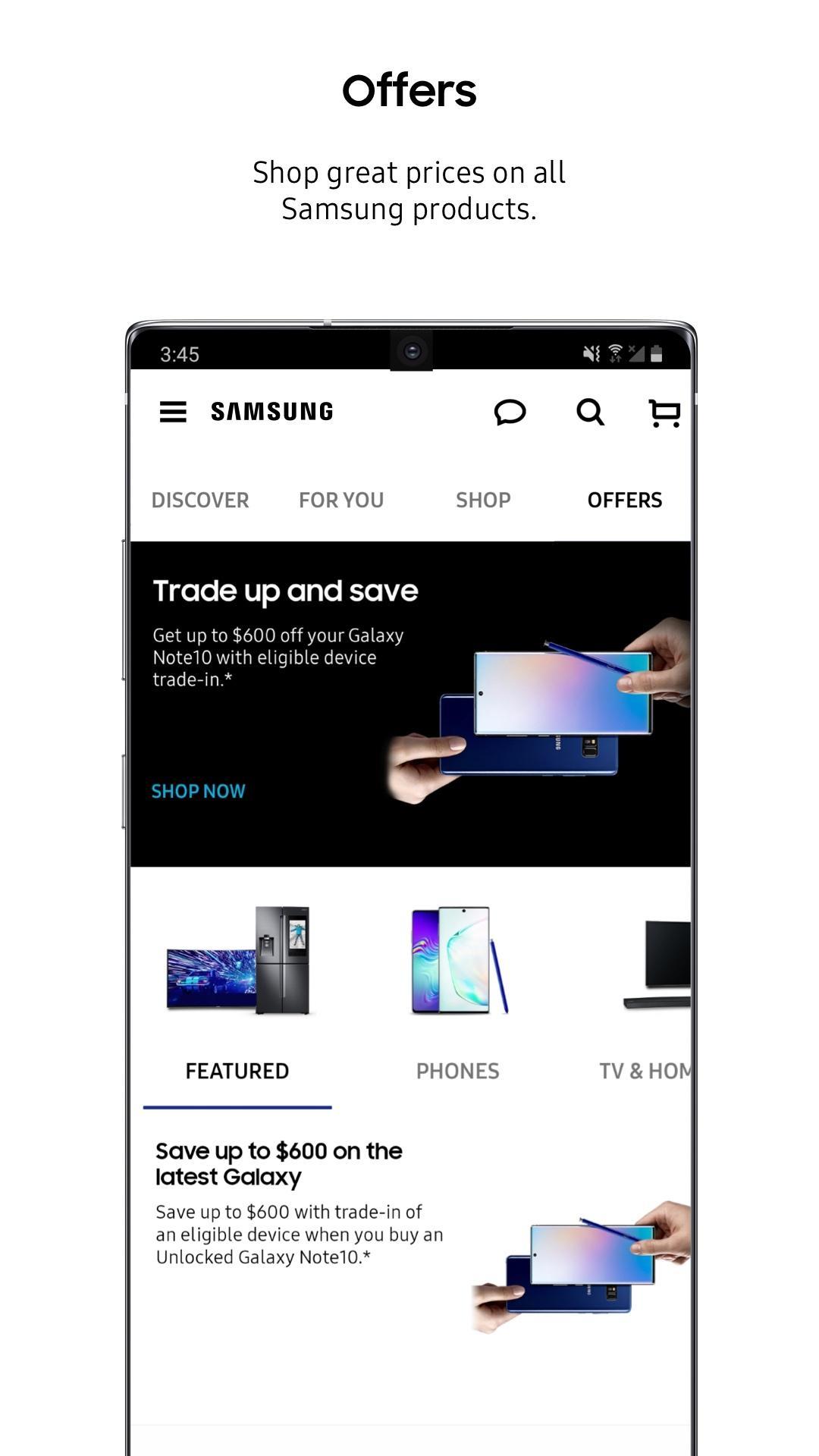This is a detailed screenshot captured from a smartphone, depicting a webpage from the Samsung website. At the very top of the image, the status bar shows the time as 3:45 on the upper left. On the upper right, typical smartphone status icons are visible, including the battery indicator, cell signal strength, Wi-Fi connection, and a Bluetooth symbol.

In the upper left corner, the word "Samsung" is displayed prominently, with three horizontal bars next to it symbolizing a menu. Adjacent to the "Samsung" logo are several icons: a speech bubble, a magnifying glass symbolizing the search function, and a shopping cart icon.

Below this header section, the first colored elements appear on the image, breaking the monochrome theme. The central focus is an advertisement with the phrase "Trade Up and Save." This section features a pair of white hands holding a smartphone, prominently showcasing both the device's screen and body. The hands are positioned to emphasize the smartphone's rectangular shape, highlighting the sleek design that Samsung is promoting in this advertisement.